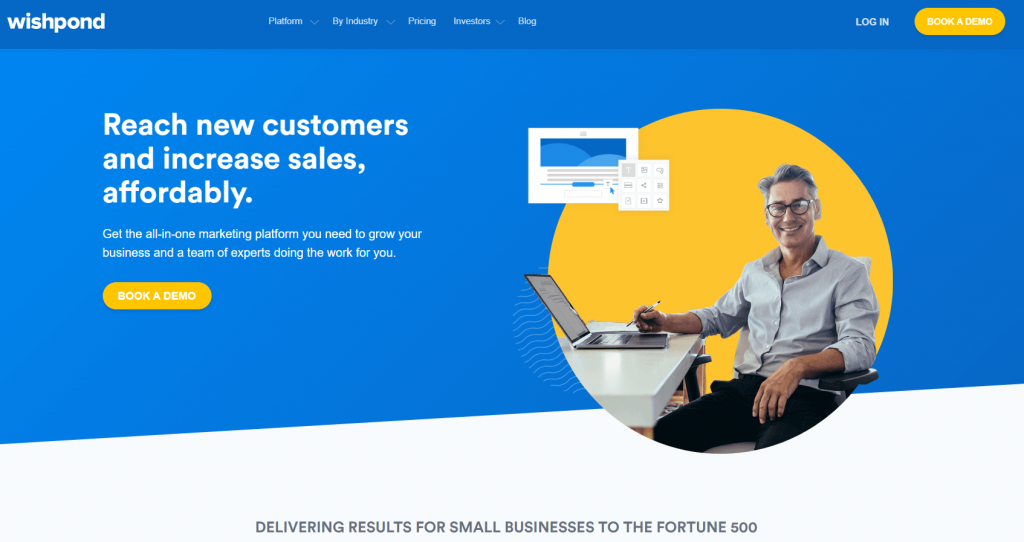**Caption:**

The image is a detailed screenshot of Wishpond's homepage. The top of the page features a dark blue header. On the left side of this header, "wishpond" is displayed in lowercase white text. Following a section of negative space, several dropdown menu options appear, each labeled in white text with a downward-facing white arrow, except for the last one. These options are: Platform, By Industry, Pricing, Investors, and Blog. To the right of these options, there is an area of substantial negative space before "Log In" appears in white text. Further right, there is a yellow button with rounded ends that reads "Book a Demo" in white text.

Below the header, the main background of the webpage is visible, dominated by a large medium blue rectangle angled slightly upwards to the right, with a light gray rectangle beneath it. In the top left corner of the blue section, large white text reads, "Reach New Customers and Increase Sales Affordably." Directly below, a smaller paragraph of white text states, "Get the all-in-one marketing platform you need to grow your business and a team of experts doing the work for you." Below this paragraph, a yellow button similar to the one in the header reads "Book a Demo."

To the right of the blue section, there is a yellow circle containing a photograph of a man at a desk. Overlaying this is a simulated screen that extends to the upper left, featuring a white background with a central blue banner and some rounded blue shapes, as well as a white pop-up window displaying a grid of icons. 

At the bottom of the gray section, dark gray text reads, "Delivering Results for Small Businesses to the Fortune 500."